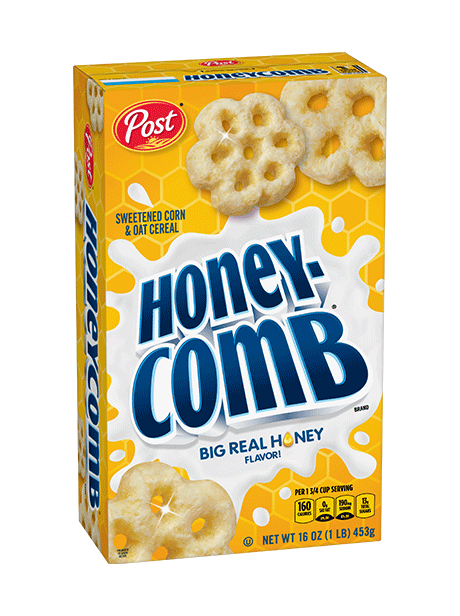The image showcases a 16-ounce yellow box of Post Honeycomb cereal. Prominently displayed in the upper left corner is the Post logo: "Post" in white letters within a red circle, outlined by a yellow border. Adjacent to the logo on the upper right, there are two large, detailed illustrations of the honeycomb-shaped cereal pieces, depicted in a lighter brown color. Another sizable honeycomb piece is placed at the bottom left of the box. In the center of the box, the brand name "Honeycomb" is written in a large navy blue font against a white splash that resembles milk. Below this, the phrase "Big Real Honey Flavor" is prominently printed in blue, with the "O" in "Honey" replaced by a drop of honey. The text "Sweetened Corn and Oat Cereal" is also included. In the bottom right corner, nutritional information and the serving size of three-fourths of a cup, alongside the calorie count, are listed in black text. The net weight of the cereal is also specified: 16 ounces (453 grams). The honeycomb theme is consistently integrated into the design, with additional honeycomb illustrations spread across the box.